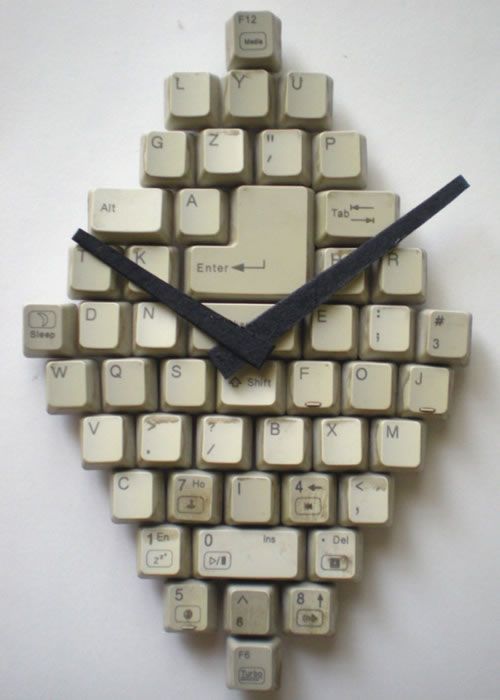The photograph is a close-up, almost artistic depiction of a makeshift clock constructed from old, dingy computer keyboard keys arranged in a diamond shape. The keys, which are discolored and range in hue from off-white to cream and gray, are lined with dirt, stains, and food remnants. They are positioned on a solid white surface, configured so that they all touch each other, forming a distinctive diamond pattern that vaguely resembles an arrow—the arrangement tapers at the top and bottom while widening at the center. Atop the diamond formation lie two black strips, possibly made of construction paper or felt, aligned like the hour and minute hands of a clock, although there is no actual clock mechanism present. The makeshift clock hands are positioned near the shift, S, and F keys, and while the keys do not spell out any specific words, they form a coherent, visually intriguing pattern that transforms mundane materials into an expressive piece of artwork.